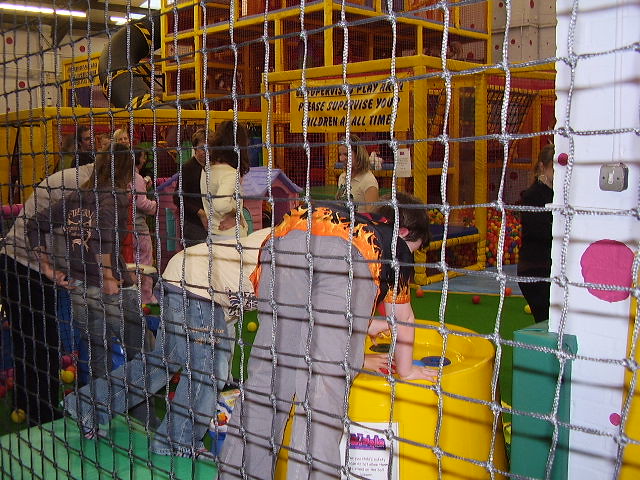The photograph captures a lively children's play area dominated by large, multi-level ball pits filled with multicolored balls. The scene is viewed through a square-gridded, dark gray net that forms a barrier in the foreground. Leaning over the net, children in blue jeans are focused on a round yellow play device. One child sports a light-colored top, while another wears a darker top with an orange flame pattern at the hem. To the left, a small group of adults watch over the activity. The background features a bright yellow jungle gym structure adorned with foam pillars and a prominent yellow banner instructing, "Please supervise your children at all times."